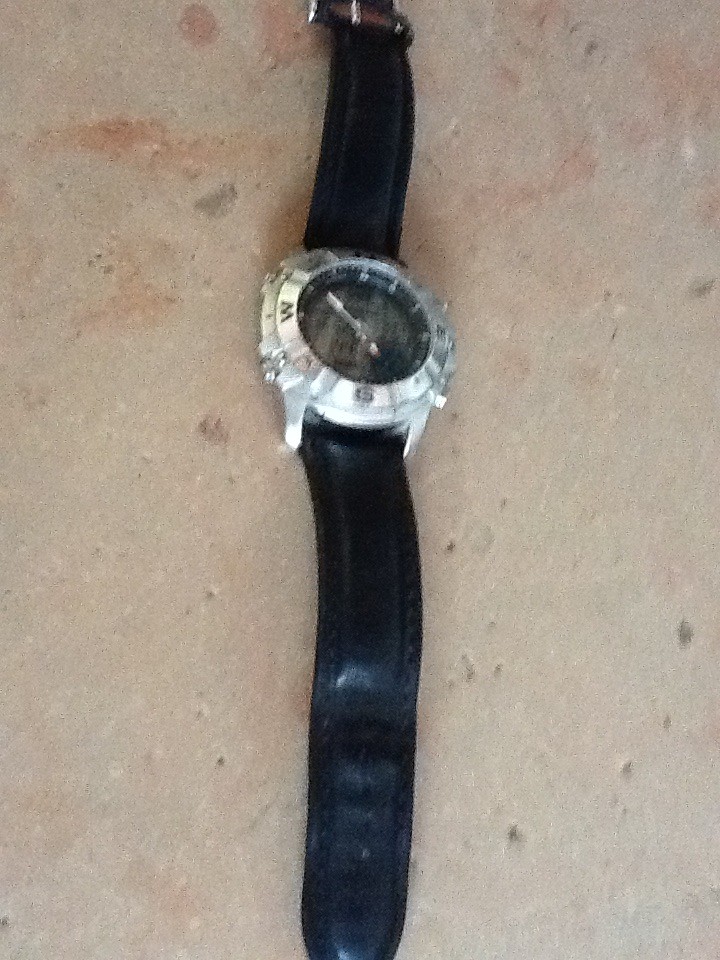The image depicts a detailed photograph of a wristwatch lying on a textured stone surface. The stone background is cream-colored, with numerous holes and scattered brown and orange flakes, contributing to a rough texture. The watch features a black leather band and a silver face. Surrounding the dial, which serves as a decorative compass, are the cardinal directions—north, east, south, and west. Inside the watch, one prominent white hand is visible, pointing at approximately 11 o'clock, though other hands are not clear. This analog wristwatch, with its intricate details and elegant design, is positioned vertically, spanning the entire length of the image.